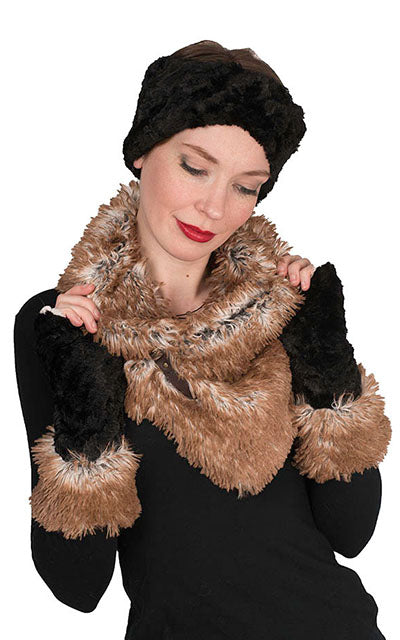The image features a Caucasian woman, seemingly modeling clothing against a plain white background. Her striking red lipstick stands out, complementing her overall look. She is adorned with a unique black headdress that resembles an open hat, revealing her brown hair underneath. The woman is draped in a sophisticated brown fur-styled scarf or jacket that gracefully rests around her arms. Additionally, she wears a sleek black long-sleeved shirt, seamlessly completing her chic ensemble.